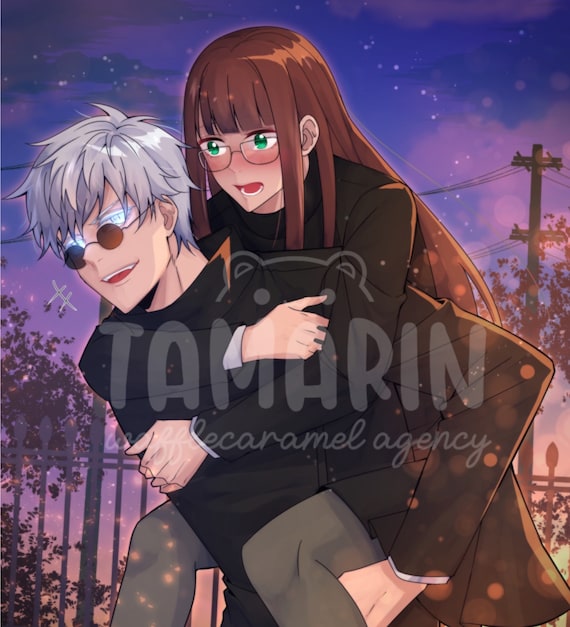In this vibrant anime-style cartoon image, we see a scene set outdoors against a twilight sky that's a mesmerizing blend of blue and purple hues, speckled with white stars. Prominent in the backdrop is a gray fence, some tree branches, electric poles with wires dangling from them, and a light pole. A watermark, barely readable, suggests it’s from the "Tamarind Agency."

Central to the image are two characters: a young woman and a man. The woman, with long light brown hair styled with bangs, sports clear glasses that accentuate her striking green eyes. She’s dressed in a black overcoat and grayish-green pants, and appears to be piggyback riding on the man. He has unruly gray hair styled in a fashionable, somewhat spiky manner, coupled with light gray, almost glowing eyes beneath small circular dark glasses hanging just below his eyes. His attire includes a black trench coat or full-zip t-shirt. Both characters have their mouths open, revealing red inside, which adds an emotional intensity to their expressions. The young woman’s arms are wrapped around the man's chest, and her legs are securely around his waist, completing her position on his back.